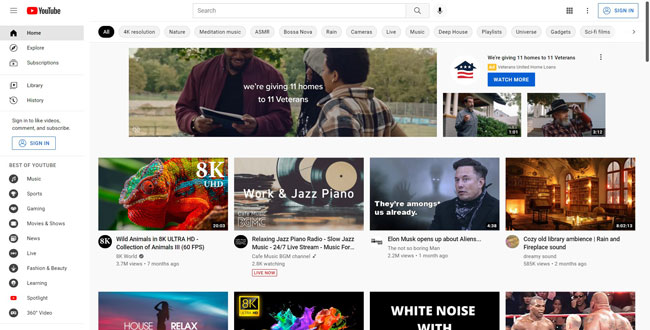This image, sourced from the website YouTube, features a detailed interface display. On the left sidebar, under the prominent YouTube logo—a white play button inside a red rectangle—there are various navigation options. These include a black "Home" button with a house icon, followed by sections labeled "Explore," "Subscriptions," "Library," and "History." Below these is a "Sign-In" button.

Further down, the "Best of YouTube" section is showcased, offering categories such as Music, Sports, Gaming, Movies & Shows, News, Live, Fashion & Beauty, Learning, Spotlight, and 360° Videos. 

At the top of the page, there is a search bar alongside another "Sign-In" button. The interface highlights content with titles including "4K Resolution," "Nature," "Meditation Music," "ASMR," "Bossa Nova," "Rain," "Live Music," "Deep House Playlist," "Universal Gadgets," and "Sci-Fi."

The main content area displays a featured video at the top, with rows of video thumbnails underneath. The first row contains three video thumbnails, followed by another row of four videos, with content continuing as you scroll down the page.